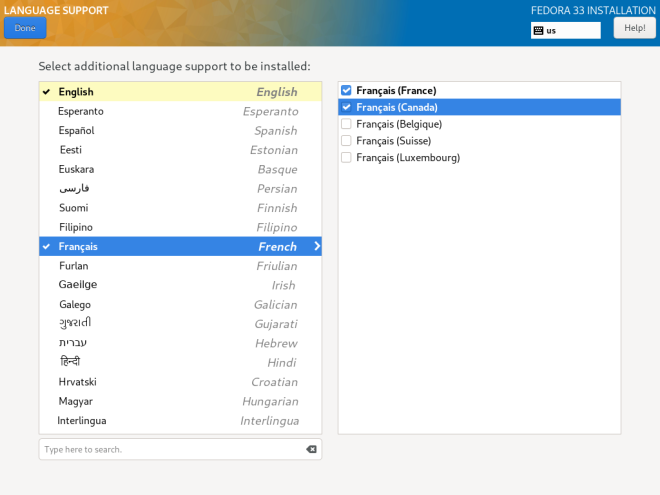**Screenshot of Fedora 33 Installation Language Support Menu**

This horizontally-oriented screenshot displays the language support menu of the Fedora 33 installation setup. The interface is divided into a main section and a top banner with a gradient design, transitioning from an orange-yellow on the left to a solid blue on the right.

**Top Banner:**
- On the left, the banner reads "Language Support" in white text.
- Positioned beneath this is a "Done" button, also in white.
- On the right side of the banner, it reads "Fedora 33 Installation" alongside a "Help" button. Additionally, there is a white box indicating "US," suggesting the current locale settings.

**Main Section:**
- The left area features a large white pop-up box containing a list of languages available for installation.
  - The heading above the list reads: "Select additional language support to be installed."
  - The first language listed and already checked is "English."
  - Further down the list, "French" is also checked, indicating it is selected for additional support. This selection is followed by a right-pointing arrow.
- A search bar is located beneath this left pop-up box, with a left arrow icon at its right end.
  
- The right area contains another large white pop-up box. This box lists specific regional variations of the selected language.
  - "France" and "Canada" are both checked, highlighting the regions for which French language support will be installed.
  - The "Canada" selection is outlined in a blue box, possibly indicating it is currently active or highlighted.

The interface design emphasizes usability with clearly labeled options and visual cues for current selections and active choices.